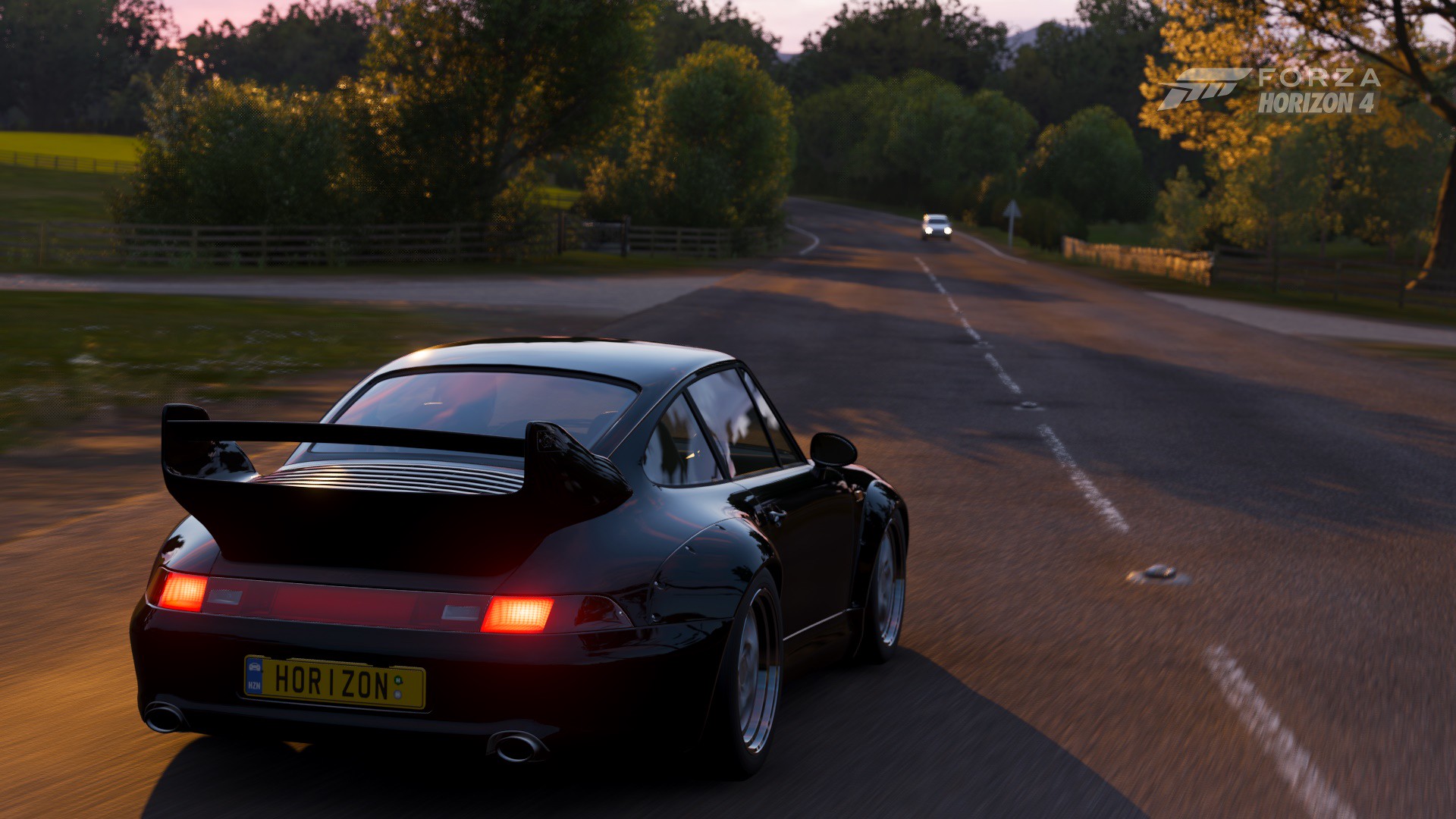This full-color photograph, taken outdoors on a street bordered by woods and a green grassy area on the left, captures the moment close to dusk or early evening as suggested by the soft sunlight. The primary focus is a black Porsche with a raised spoiler, located on the left side of the road. The car's vibrant red taillights and yellow license plate reading "Horizon" are prominently visible. The scene includes a dashed white line running down the center of the street and a white vehicle with headlights on approaching from the distance in the right lane. In the upper right-hand corner, there is text indicating "Forza Horizon 4." Surrounding the road are tall, leafy trees, adding to the natural ambiance of the setting, and a triangular traffic sign is partially visible behind the Porsche, indicating a nearby turn-off.